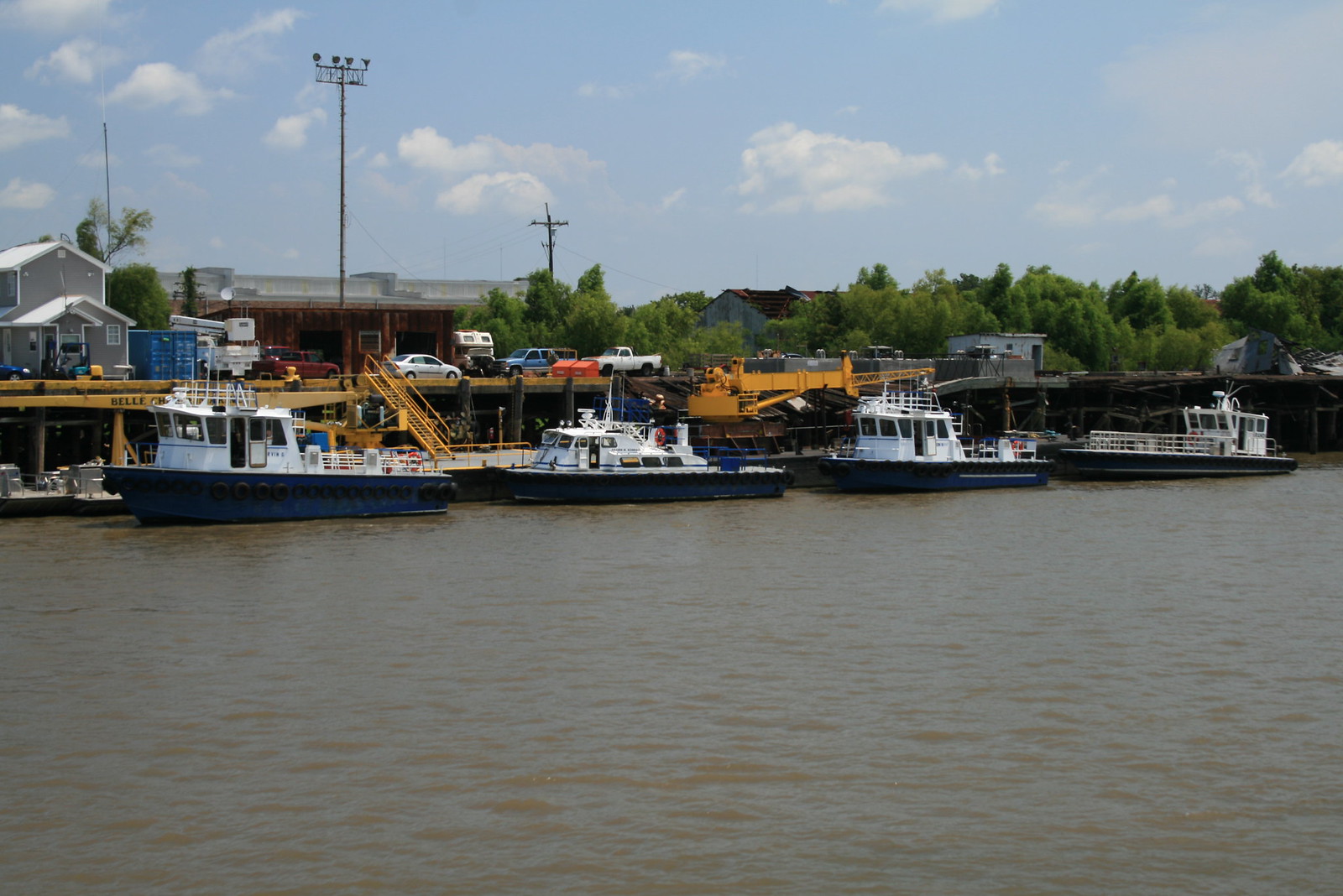The image depicts a vibrant, bustling harbor scene. In the foreground, four small trawling boats or possibly police boats, distinguished by their white cabins and navy or black underbellies, float on murky, brownish-gray water. A bright yellow ladder descends from the dock to the water's edge. The dock itself, clearly a working dock, is populated with cars and machinery, including a striking orange crane and bright yellow stairs leading up to a parking lot. To the right, a line of lush green trees stretches behind the boats, with several tree houses nestled among the foliage. Further in the background on the left side, there’s a yellow elevated bridge bustling with vehicular activity, flanked by maintenance buildings. Above, a serene light blue sky is dotted with fluffy white clouds, providing a peaceful contrast to the industrious scene below. The entire harbor is enveloped in a lively yet functional atmosphere.